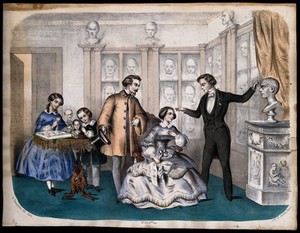The illustration depicts a room reminiscent of an old-fashioned or Victorian-era setting, filled with statues and busts, suggesting it may be a sculptor's showroom. The room is elegantly decorated, with a distinct yellow curtain draped above adding to the ambiance. Multiple display cabinets showcase various busts, while a pedestal to the right features an intricate design carved with figures, supporting a prominent bust.

To the left, an open doorway leads into another space, highlighted by a blue carpet. The scene includes five people: a young girl in a blue dress and a boy in black attire stand to the far left, seemingly engrossed in viewing something. Nearby is a man in a brown overcoat, who directs his attention towards the seated woman in an elaborately flowing gown. This woman, positioned near the center, gazes at a bust beside her. At her side stands a man in a black suit, possibly demonstrating or discussing the statue with her. The muted, formal colors and detailed attire of the individuals suggest they are part of a sophisticated gathering, possibly evaluating or appreciating the artwork displayed around them.